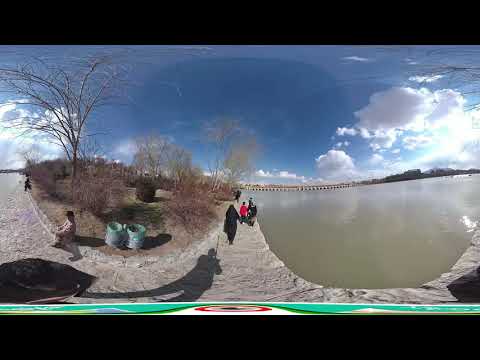A striking outdoor photograph captures a tranquil park or recreational walking area beside a calm lake or large pond. The scene is dominated by vivid, blue skies filled with puffy white clouds, and bright, natural light filtering through. On the left side, a curved stone walkway starts at the image's center horizon and winds its way to the forefront, leading to the right. This walkway, with its beige-grey cobblestones, is populated with several people strolling along its path. Notably, a young boy, around seven or eight years old, sits on a low stone wall by two trash cans near the walkway's curve.

A prominent, leafless, brown tree stands just behind the boy, indicating a late fall or winter setting. The surrounding vegetation also appears barren and brown, contributing to the seasonal atmosphere. On the right side, the murky, reflective waters of the lake stretch from the center of the image to the edge, framed by the walkway. A woman, clad in a full black outfit with only her eyes visible, walks near the dam-like structure, suggesting the photo's possible Middle Eastern location. The fisheye lens has caused a slight distortion, giving the image a unique perspective. The shadow of the person taking the photograph extends prominently across the cobblestone walkway, adding a human touch to this serene landscape.